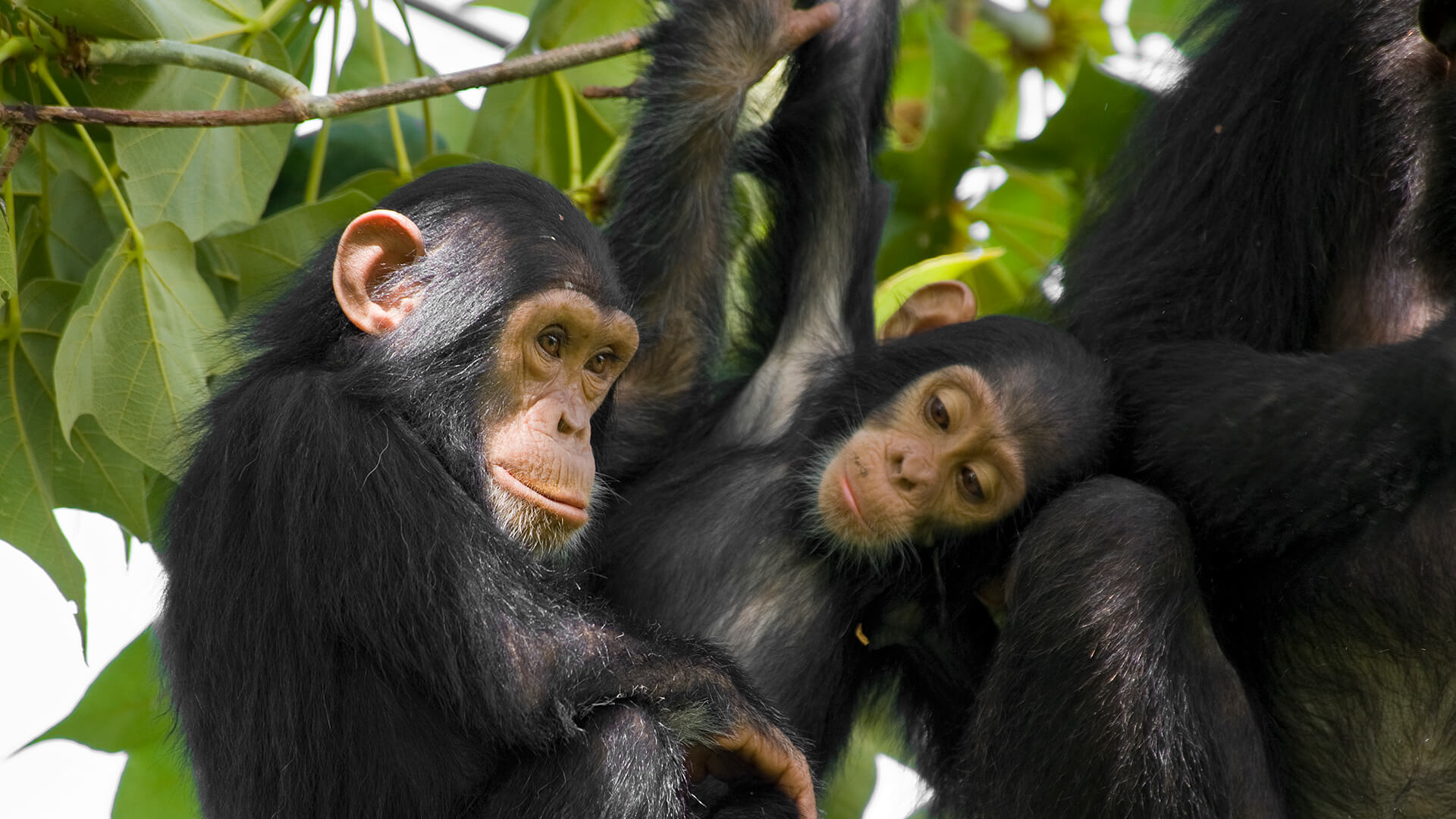In this detailed close-up color photograph, we observe a trio of chimpanzees intimately positioned on a lush, leafy tree. The left side of the image features a slightly larger chimpanzee gazing to the right, its ear visibly illuminated by a ray of sunlight. This chimpanzee, appearing protective, holds a juvenile chimp by the waist. Positioned centrally, the younger chimp seems almost nestled in the lap of the larger one, directing its gaze slightly downward with its head angled to the left. The detailed texture of their black fur is clearly visible. On the right-hand side, partially cropped out of the frame, is a glimpse of a third, presumably larger, chimpanzee, identifiable by part of its body and leg, but with its face unseen. The background displays an abundance of large, deep green leaves on long stems, effectively conveying the dense foliage of their arboreal habitat. The chimps appear calm and relaxed, captured in a serene moment amidst the verdant expanse of the tree.